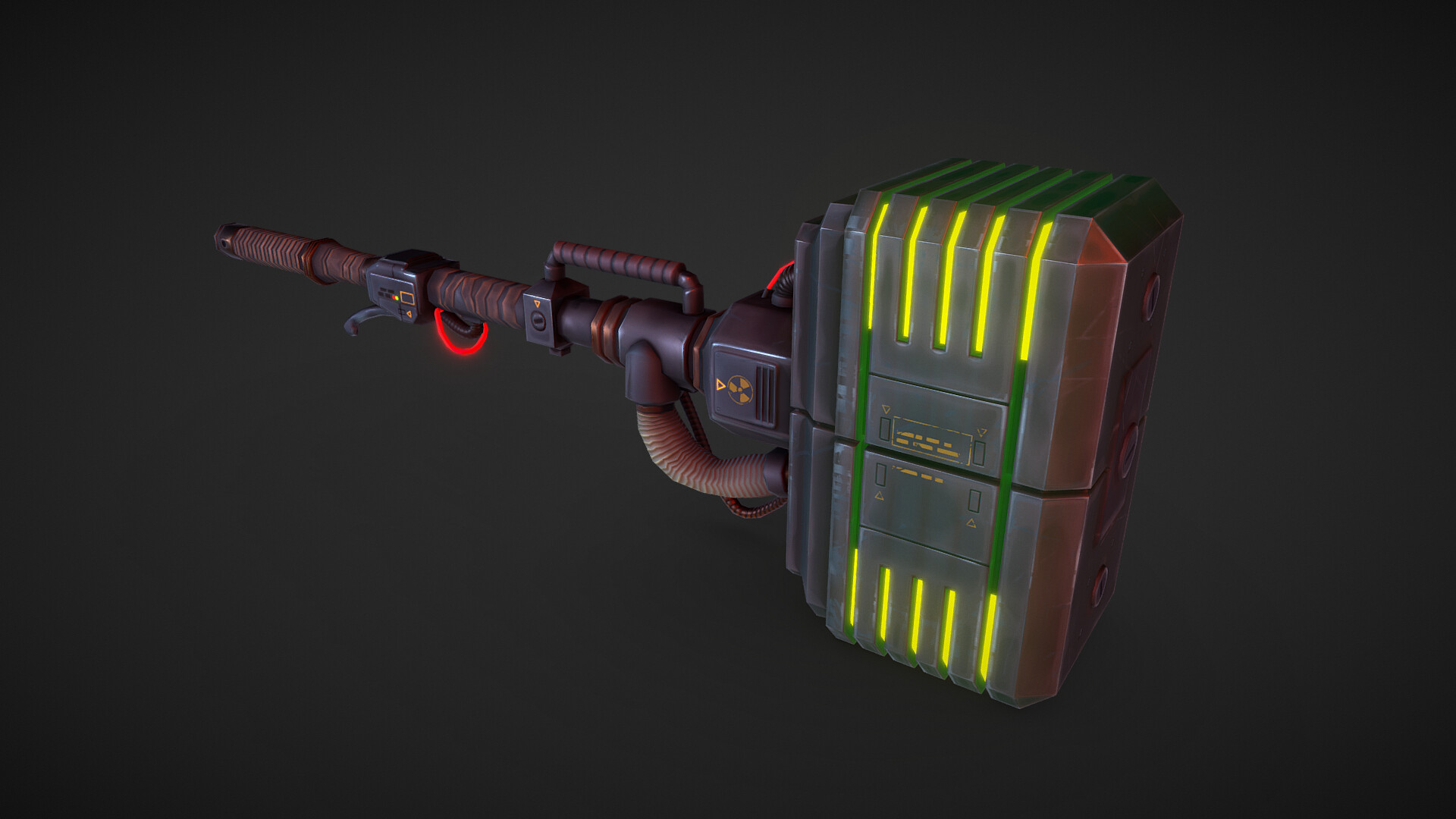The image features a 3D modeled, electrically-powered, sci-fi hammer highly reminiscent of designs seen in PS3 or PS4 games. The hammer stands out against a plain, gradually darkening gray background. At the very right, the hammer's head showcases a brownish top with unreadable, raised scribbles. The sides of the hammer's head are adorned with striking yellow and green neon lights, and a radiation caution symbol embellishes the base, hinting at its nuclear capabilities. The handle is a sophisticated assembly of copper tubes and bolts, interspersed with intricate wiring that suggests its electrical nature. A distinct feature is the segmented handle design, which includes tube sections alternating with square sections, further emphasizing its futuristic look. The hammer also features a raised bar handle for side or base grip, enhancing its practical design.